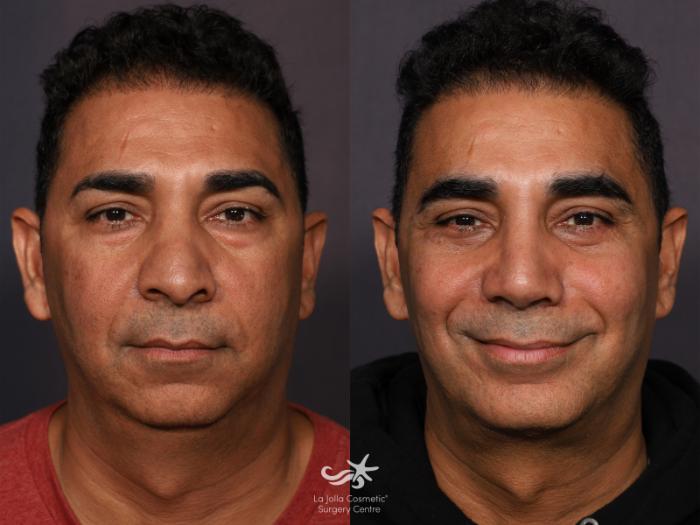This is an image featuring two side-by-side photographs of the same man, showcasing a potential before-and-after transformation. Both images have a similar gray background, with the one on the left being slightly darker. In the left photograph, the man has short black hair, styled slightly upward off his forehead, with dark, bushy eyebrows, and brown eyes. He is wearing a red t-shirt and has a neutral expression, without any clear emotional indication. There is a subtle shadow suggesting a five o’clock shadow on his mustache area and possible scars on his forehead.

In the right photograph, the man is smiling broadly, though not showing his teeth. His hair appears a bit longer and higher on the top. He still has the same dark eyebrows and eyes, and he's wearing a black t-shirt with an additional shirt or hoodie over it. The background remains the same gray tone, maintaining consistency between the two photos. He seems noticeably happier, and there might be an implication of some work done on his chin or neck, suggesting a cosmetic transformation.

Central to both images is a watermark at the bottom, with the logo featuring a star with wave patterns and the text "La Jolla Cosmetic" in gray, indicating the possible involvement of a cosmetic company in the depiction of these changes. The man’s consistent features across both images – such as his hair, eyebrows, eyes, and overall facial structure – reinforce that it is the same person in different emotional states or possibly before and after a cosmetic procedure.